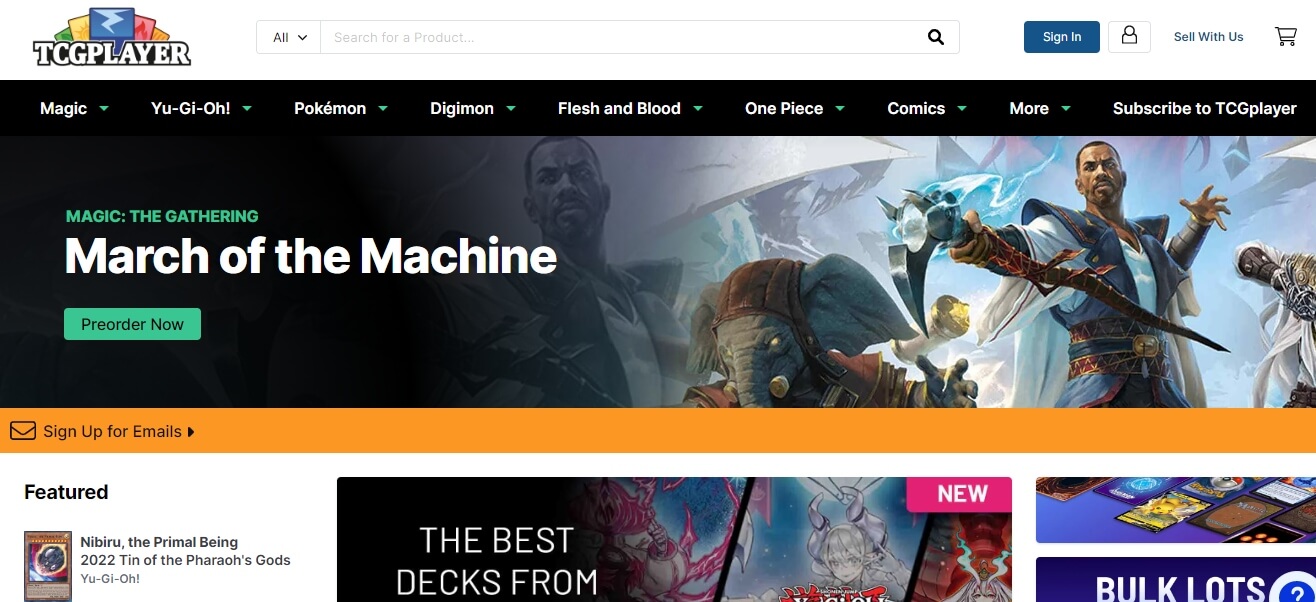The screenshot is of a website titled "TCG Player," prominently displayed in the upper left corner. At the very top of the page, there is a search bar, and the upper right corner features options to "Sign In," accompanied by a small profile icon. Adjacent to these options are links to "Sell With Us" and a cart icon for shopping.

The website features multiple tabs, including "Magic," "Yu-Gi-Oh," "Pokemon," "Digimon," "Flesh and Blood," "One Piece," "Comics," "More," and a final tab labeled "Subscribe to TCG Player."

The header image showcases promotional text for "Magic the Gathering: March of the Machine" with an invitation to "Pre-Order Now" highlighted in a prominent manner. Below the header is an orange banner urging users to "Sign Up for Emails."

On the left side of the page, there is a section titled "Featured," highlighting a Yu-Gi-Oh card named "Nibiru, the Primal Being" from the "2022 Tin of the Pharaoh's Gods." Below this section is a partially cropped heading that begins with "The Best Decks From..."

On the right side, a small image depicts what appears to be the back of several trading cards. Adjacent to this is another image featuring the text "Bulk Lots," though the rest of the content in this image is also cropped out.